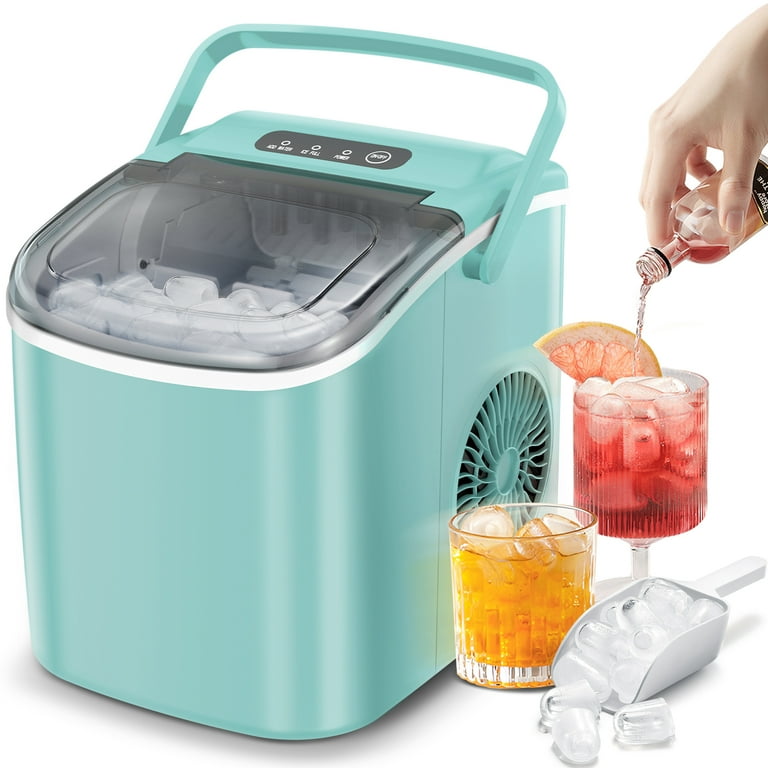The promotional image showcases a contemporary, portable ice maker in a sleek cube shape with rounded edges. The appliance is an eye-catching teal or seafoam green color, complete with a matching handle on top. The top area features a digital keypad interface, though the specific settings are not legible. Through a transparent plastic window on the top, one can observe ice being made inside. The scene is well-composed, highlighting two glasses filled with ice beside the machine—one containing a yellow drink, possibly with a slice of lemon or orange, and the other with a red beverage, which a hand with manicured nails is pouring into the glass. Additionally, an ice scoop filled with ice is placed in the bottom right corner of the image, reinforcing the utility and modern elegance of the appliance.